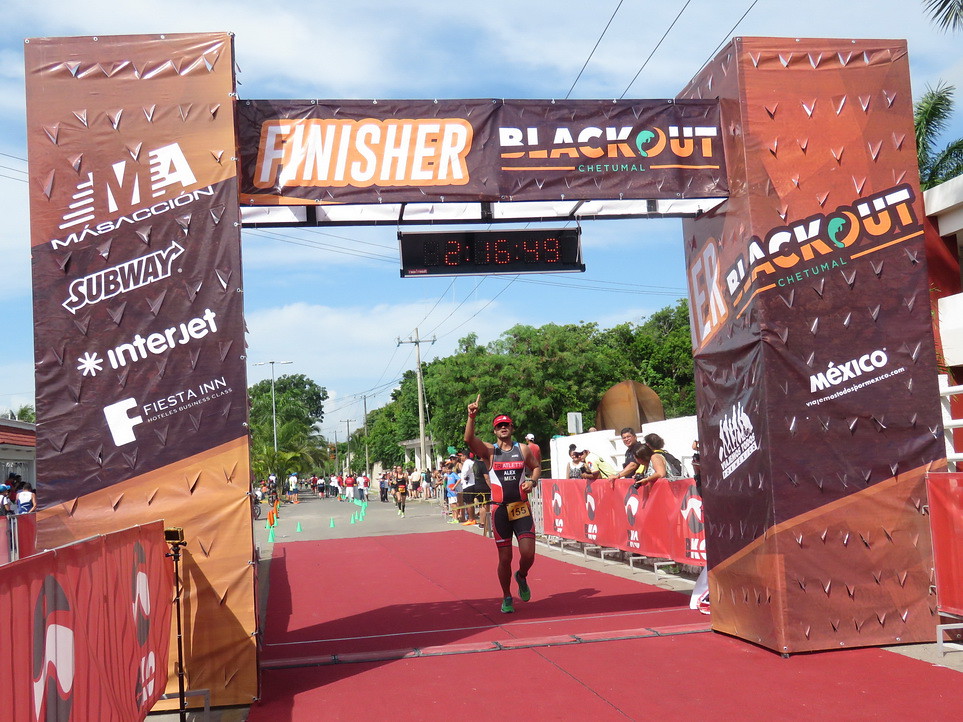The photograph captures the exhilarating moment of a racer nearing the finish line of a sunny marathon. The race takes place on a street dotted with palm trees under a sky with thin wisps of clouds. Dominating the scene is a large, square arch constructed from plastic banners in shades of brown, rust, and orange. The arch is emblazoned with the words "Finisher" and "Blackout, Chetomal" in white and orange letters. Suspended beneath the arch is a digital clock, brightly displaying a race time of 2:16:49.

The runner, wearing a black and red outfit accented with white, along with a red visor, raises his right hand, pointing a finger triumphantly as he almost crosses the finish line. A red carpet runs beneath his feet, adding to the vibrant atmosphere. His runner’s number is clearly visible, and he sports red baseball cap, green shoes, and a tank top paired with shorts. In the background, more runners can be seen approaching, with spectators lining the street, leaning over the barriers to cheer him on.

The archway itself is supported by two wooden beams, each wrapped in advertisements for brands like Blackout, Chetomal, Mexico, Subway, Interjet, Fiesta Inn, and Mesa Coin. The scene is a lively snapshot of determination, support, and celebration amidst the final moments of the race.